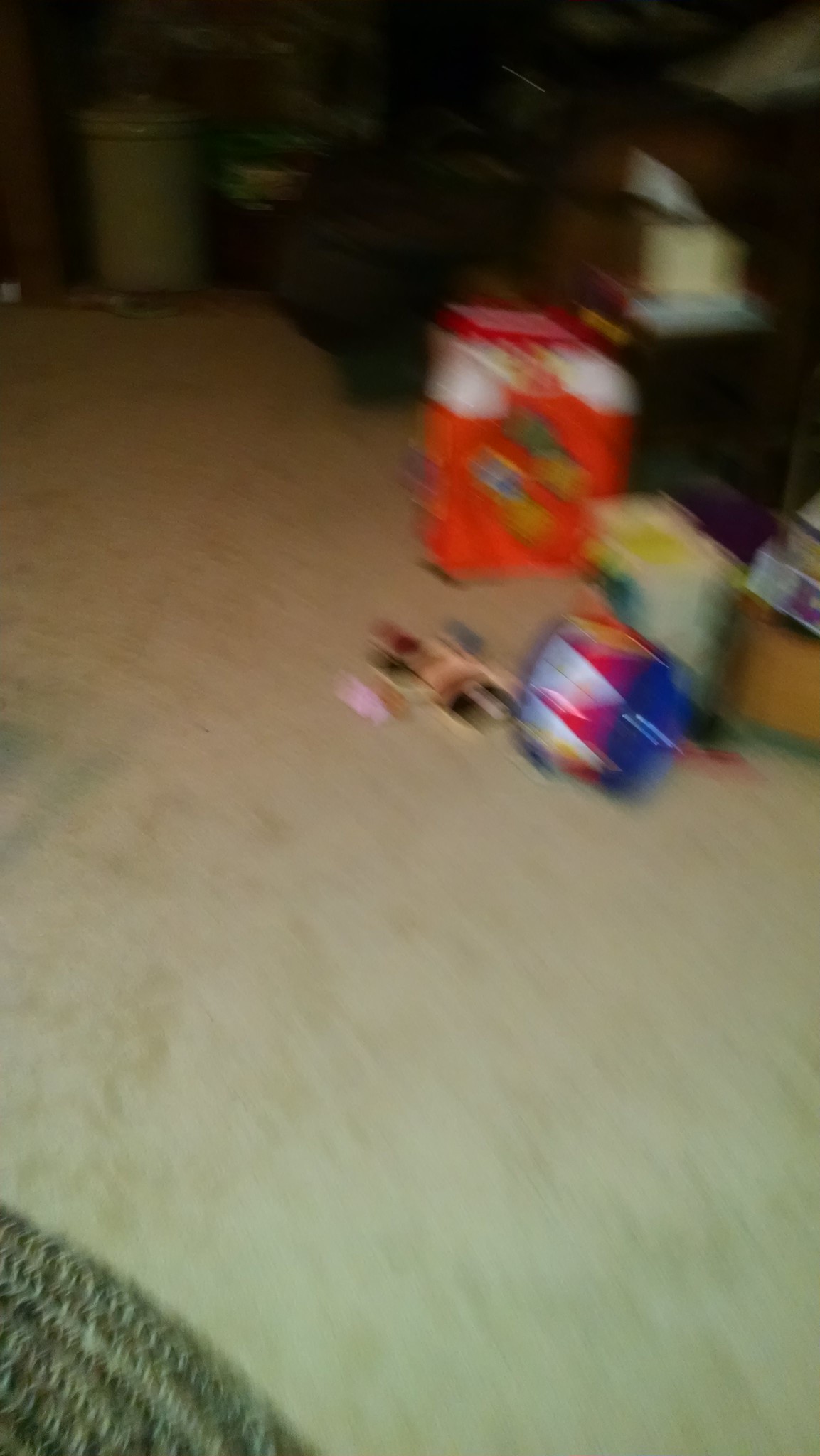This extremely blurry photograph appears to be taken inside a dimly lit room in a house. The back of the room is almost completely obscured in shadow and further blurred, making the furniture silhouettes indiscernible. The floor, which seems to be a light gray or off-white, possibly beige, is mostly hidden due to the blurriness of the image. In the front left corner, the edge of a round, plain greenish-gray knit rug is visible. Scattered on the floor are a few children’s toys, including a plastic toy drone near a sideways blue and pink drum, accompanied by other indistinct objects. The room also contains some indistinct tan and pink items, possibly another toy or a piece of furniture, along with a suspected trash can towards the back.